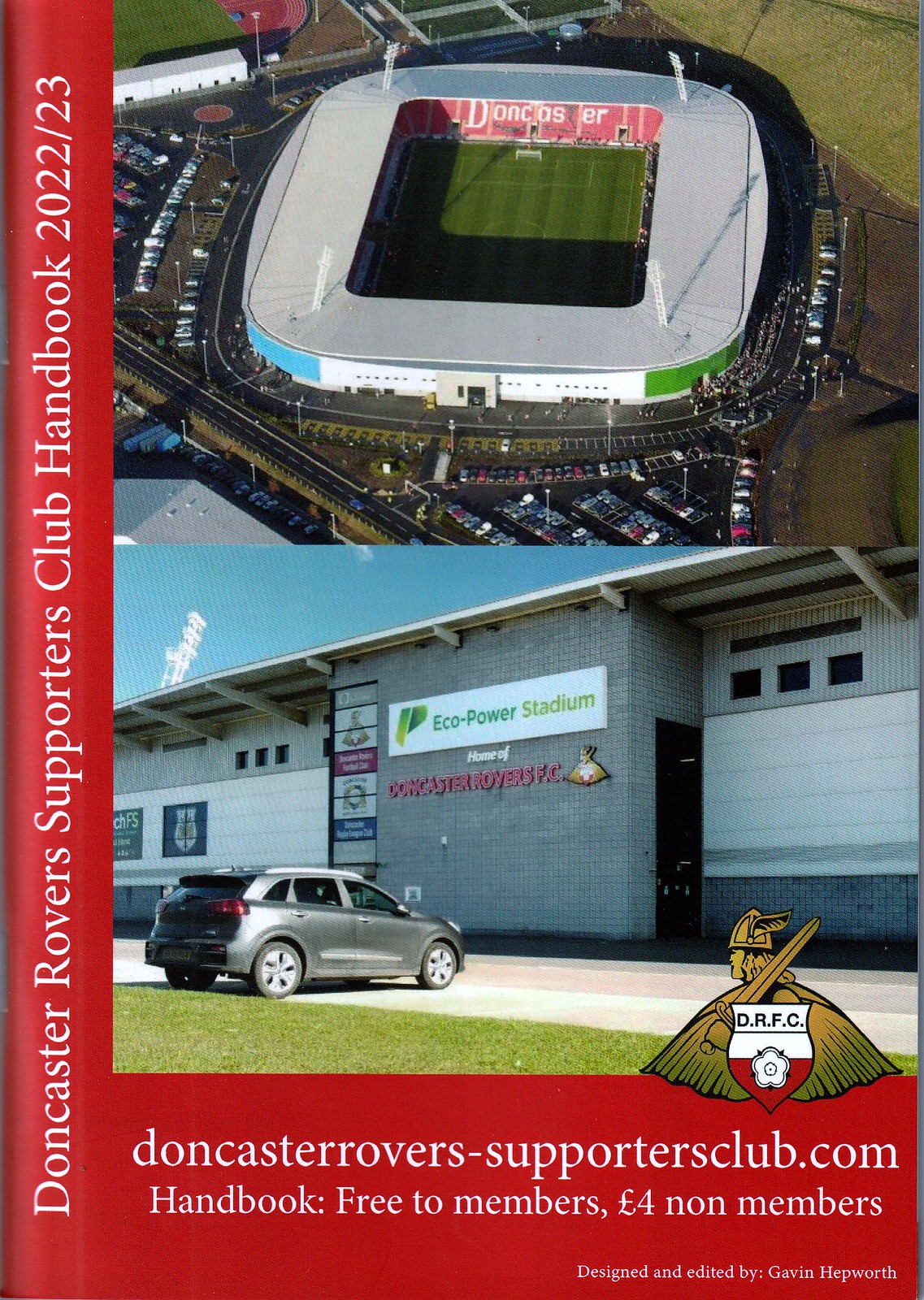The split image showcases two distinct visuals. The top half is an aerial photograph of an open-air soccer stadium, identified as the Doncaster Rover Sports Club, with visible grassy infield, red seating, and a parking lot filled with cars. The stadium is viewed through an opening in the roof, capturing the essence of the venue. The left side of the image features a red border with the text "Doncaster Rover Supporters Club Handbook 2022-2023" in white.

The bottom half of the image shows a car parked in front of a garage door or an entrance to the stadium, labeled "Ecopower Stadium." The DRFC emblem, depicting a Viking with a sword on his shoulder, is also present. At the bottom, the text "DoncasterSupportersClub.com Handbook, free for members and £4 for non-members," underscores the advertisement's motive, emphasizing it as a promotional material for the Doncaster Supporters Club. The image includes colors such as red, white, green, gray, blue, and black, creating a dynamic and vibrant presentation.